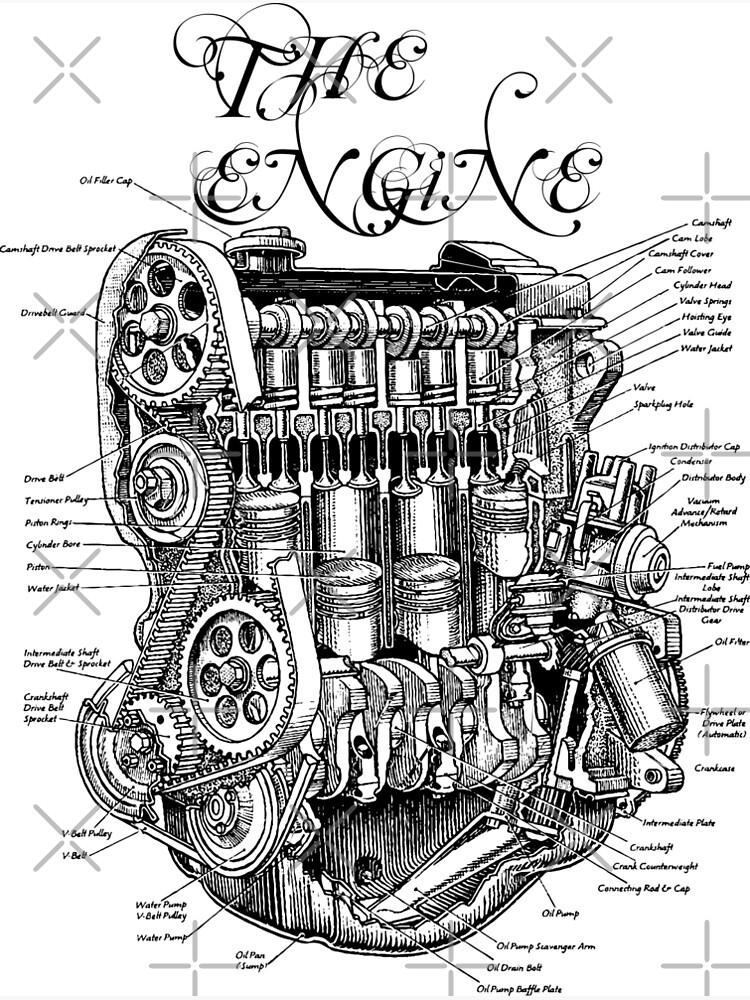This black and white illustration, reminiscent of an old-fashioned engraving, provides a detailed diagram of an engine. At the top, in a fancy script, the image is titled "The Engine." The roughly square-shaped engine compartment is meticulously depicted, showcasing various components in a digital drawing set against a white background. The left side of the engine features numerous gears connected by a belt, while the middle section prominently displays the pistons and crankshafts. The right side houses circular and cylindrical elements. Annotative lines extend from different parts of the engine to corresponding labels, identifying numerous components such as the camshaft, valve springs, cylinder head, oil pump, and flywheel. Some labels, rendered in black lettering, are less legible, while others clearly identify parts like the ignition distributor cap, condenser, and fuel pump. Gray Xs and crosses scattered throughout the image suggest an attempt at copyright protection.